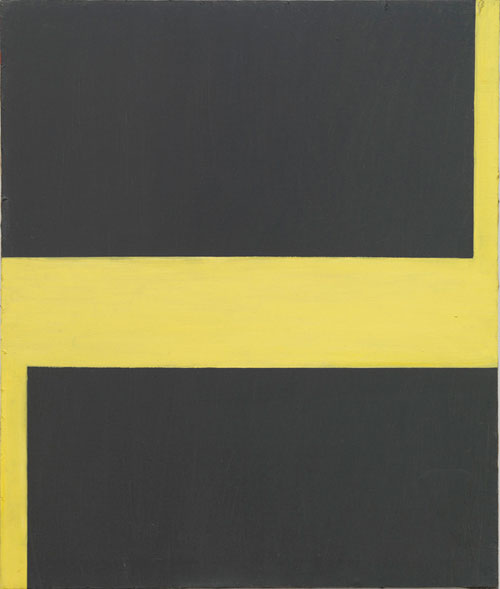This modern painting features a striking contrast of black and yellow hues. Dominating the composition is a vibrant yellow shape resembling an angular, deconstructed chair or a zigzagging "Z" turned on its side. The yellow form begins as a rectangular block at the bottom of the image, extends upward to the center, and then broadens into a horizontal stripe crossing to the right edge. From this point, it continues vertically upward along the right border of the image. The entire background is a deep, uninterrupted black, providing a stark backdrop that accentuates the geometric yellow design. The image does not contain any text or additional colors, maintaining a minimalist yet compelling aesthetic focused solely on the interplay of these bold shapes and contrasting colors.